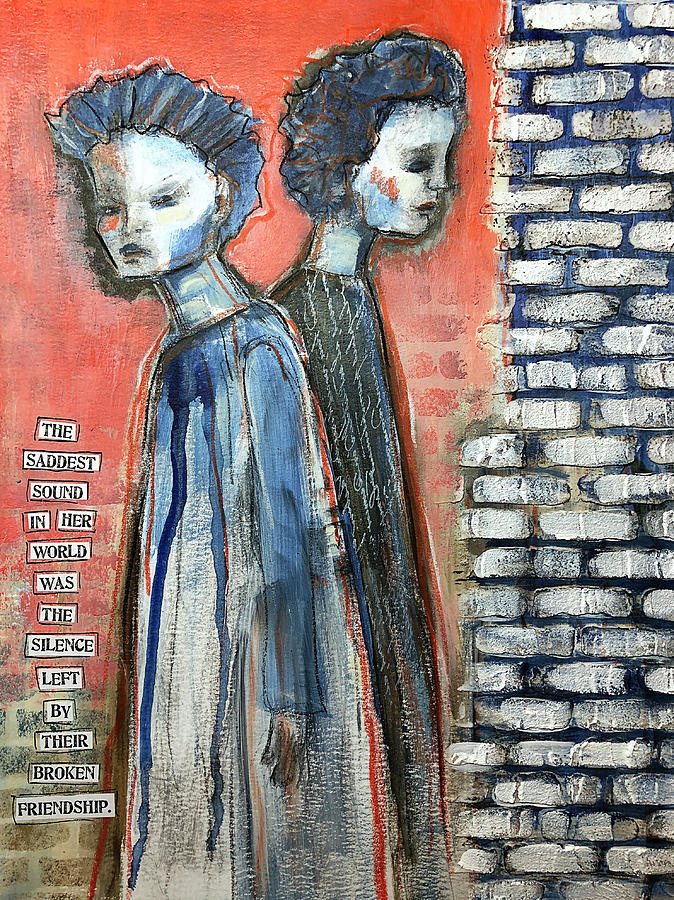This detailed artwork showcases an emotional scene with two female figures, captured in an eerie, possibly emo style. The background features an orange gradient, dark at the top and gradually fading to light at the bottom. On the right, there is a white brick column with navy blue grout, resembling a fireplace chase. The woman on the left, with a serious expression and light still in her eyes, wears a flowing off-white and blue dress with a single red streak. She gazes directly out at the viewer, her hair styled away from her face. The woman on the right, with hollow, black eyes and curly hair, stares off to the side, her frame appearing notably thin. She dons a long, glamorous, black dress adorned with cursive writing. The accompanying text, situated to the left of the image, reads: "The saddest sound in her world was the silence left by their broken friendship," emphasizing the melancholic tone of the piece.